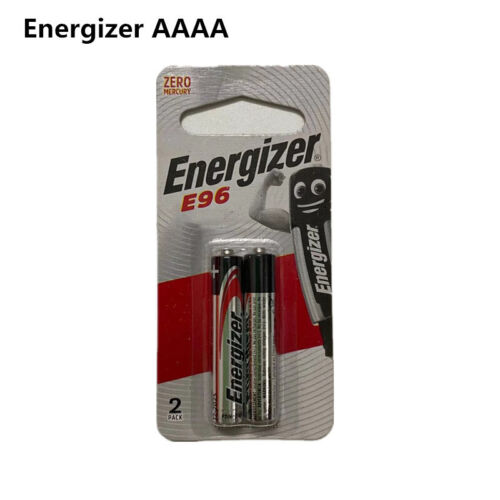An image displays a two-pack of Energizer E96 batteries encased in clear plastic packaging. Prominently situated beneath the cutout for the hanger, the "Energizer" brand name is featured in bold black lettering, occupying the top third of the package. The "E96" labeling is highlighted in bright red. Below the two visible batteries, there is a broad red bar design. Centrally located on the right side of the package is the Energiizer logo, depicted as a cartoon Energizer battery, complete with eyes, a smiling mouth, and a right arm raised in a fist. In the top left corner, "Zero Mercury" is prominently printed in red lettering. The bottom left of the packaging confirms this is a two-pack. The batteries themselves retain the traditional Energizer design: a silver body with black lettering and a black band at the top, accented by a red design along the left side.